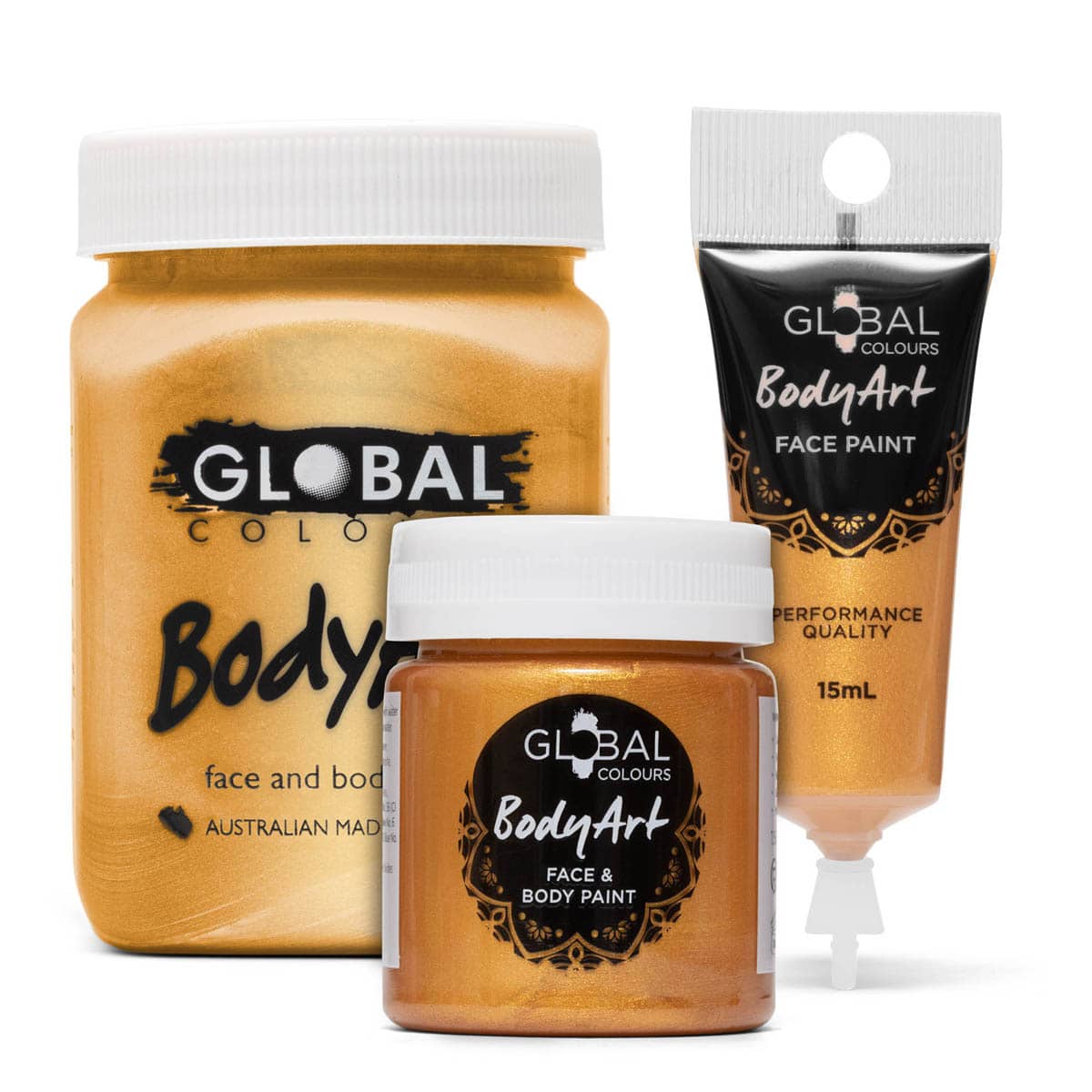The image showcases a collection of beauty products from the Global Colors brand, specifically their body art paints. On the left, there is a large jar with a yellowish-brown body and a white screw-on lid, labeled "Face and Body." In front of it, there is a smaller jar with a darker brown body and a similar white lid, marked as "Face and Body Paint." To the right, there is a tube with a black and brown body and a white cap, labeled "Face Paint." All containers feature the Global Colors branding and are noted for their performance quality. The products exhibit a cohesive design with white lids and black or white lettering detailing their use for face and body painting. The paint itself is visible as a gold or orange liquid, reflecting a vibrant hue suitable for various body art applications.